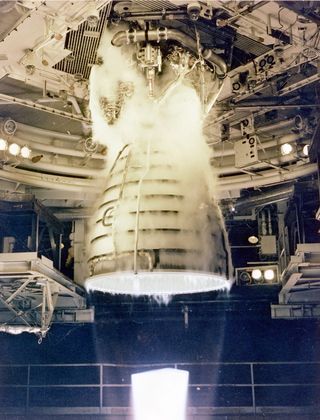This photograph captures the intricate undercarriage of a rocket during what appears to be a test or launch sequence. The focal point is the rocket's engine, a prominent metal cone at the center, emitting a glow with hints of fumes and fire beneath it. Surrounding the engine, the rocket’s undercarriage reveals an off-white to beige color scheme, adorned with numerous metallic rings, grates, and circular black components likely acting as vents. Also visible are an array of large silver pipes or vent systems, adding to the complexity of the machinery.

The setting hints at an industrial or manufacturing plant, evidenced by the presence of various equipment, safety rails, and an intricate network of wires and pipes on the ceiling. A large cone-shaped light hangs overhead, surrounded by fog, suggesting the room's cold atmosphere. A background fence and rails for safety further reinforce the industrial nature of the site. Overall, the image conveys the sophisticated and high-tech environment required for rocket technology, emphasizing the engine’s powerful and active state amidst a backdrop of detailed, utilitarian infrastructure.